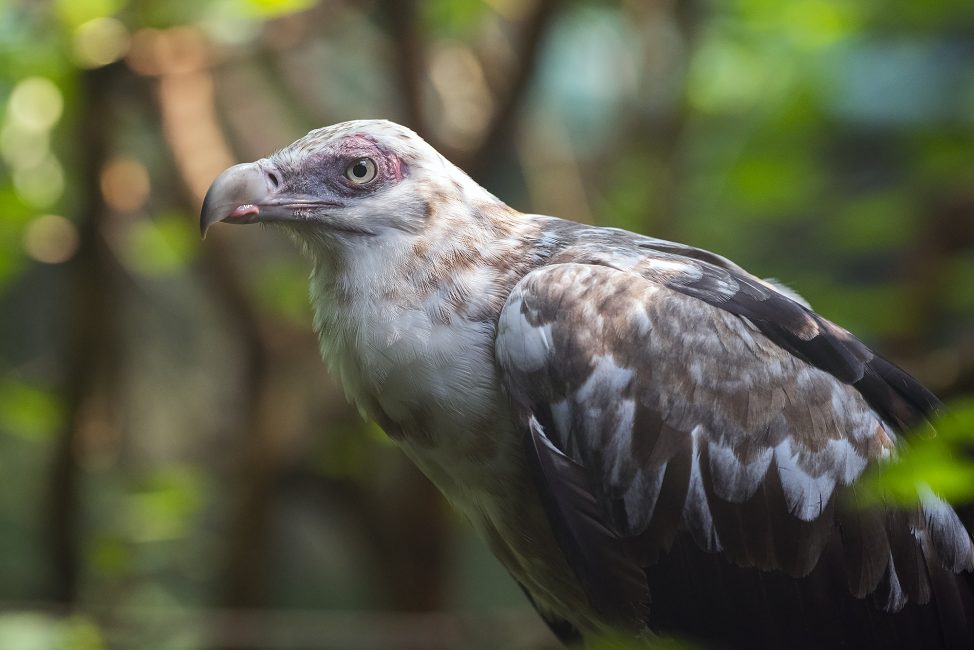The image captures a large bird, possibly an eagle or a hawk, with a strong and focused composition. The bird is depicted in profile, facing the left side of the frame, showcasing its powerful presence. Its beak, which is light brown to grayish in color, curves sharply downward into a spike, suggesting it is a predator, potentially a meat eater. The eye, which appears black with a distinctive slash-like marking above it, enhances the bird's intense, aggressive look. The feathers around its head are predominantly white with streaks of gray, transitioning into darker shades as they extend downwards. The bird's wings exhibit a mix of grayish, brown, and white feathers, and its body shows these colors intermingled. The background is heavily blurred, featuring varying shades of green, which emphasizes the depth of field and ensures the bird remains the focal point of the image. Additionally, it seems there might be something in the bird's beak, though it is not entirely clear what it is. The bird's poised and striking demeanor is accentuated by the photograph's detailed rendering of its feather patterns and color transitions.